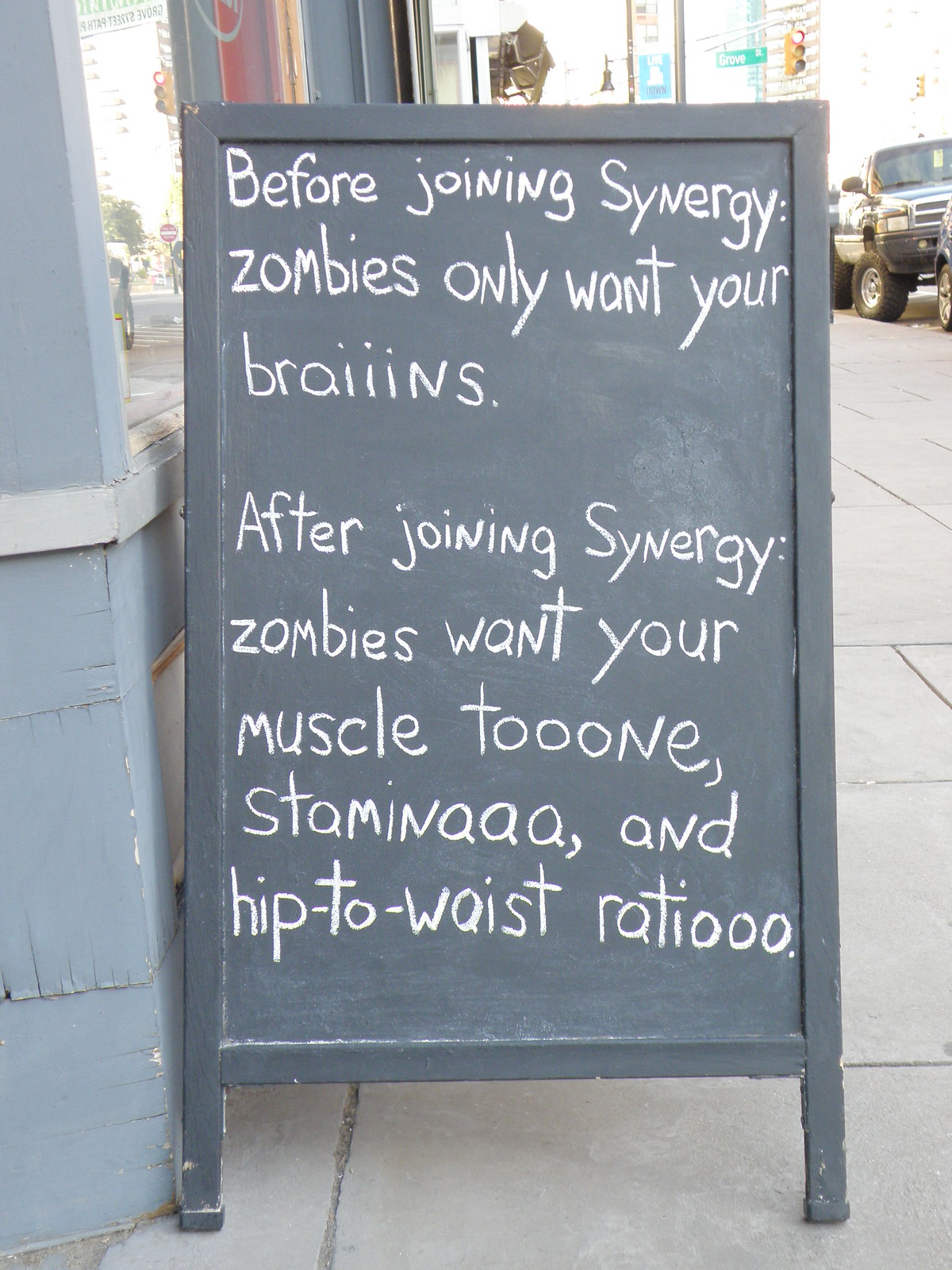This photograph depicts a chalkboard sign positioned on a city sidewalk, outside a building with faded blue paint. The gray board, written in white chalk, contains a humorous message about a fitness center named Synergy. The sign reads: "Before joining Synergy: zombies only want your braiiins. After joining Synergy: zombies want your muscle tooone, staminaa, and hip-to-waist ratiooo." The mispelled words add a playful touch. Concrete squares form the sidewalk while, in the background, a blue and white pickup truck, likely a Dodge, is parked. There's also a stop sign with a red light and a green street sign visible in the distance. The day appears to be clear and sunny, with a noticeable glare in the upper right corner. This comedic sign aims to encourage people to improve their fitness for the hypothetical approval of zombies.